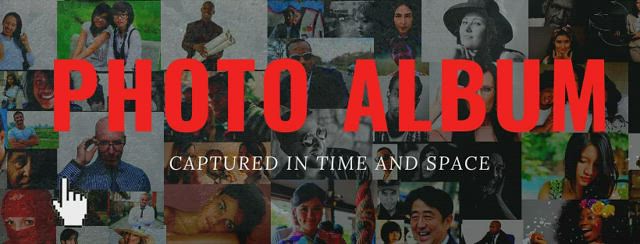This landscape image is a wide rectangular photo album cover, featuring a grid-like collage of various pictures in the background. These photographs depict a variety of subjects, including women, men, friends together, and people in different poses such as lying down and looking down. The images are diverse, showcasing different races, ages, and backgrounds, with some in black and white and others in color, arranged in various shapes and sizes including squares and rectangles. Prominently across the middle of the image in bold red letters is the text "Photo Album," and beneath it in smaller, non-bold white text are the words "captured in time and space." In the bottom left-hand corner, there is an icon of a right hand with the thumb and pointer finger extended, the remaining fingers bent, pointing upwards. This detailed collage emphasizes the theme of capturing moments and diverse experiences across time and space.